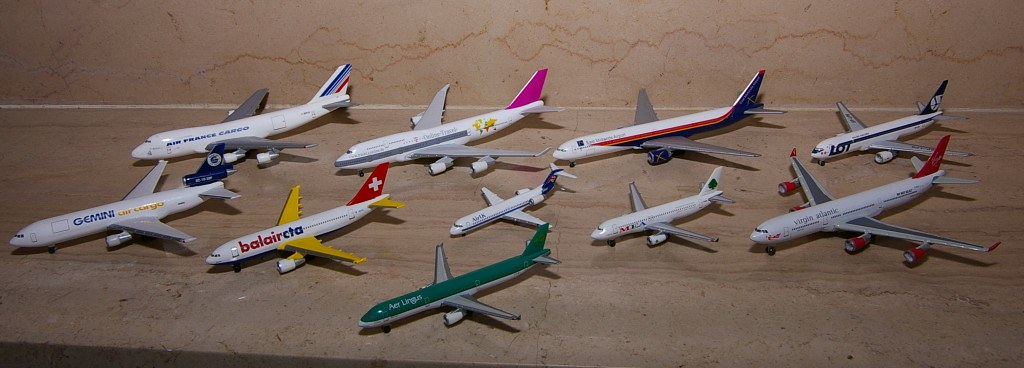The photo captures a detailed collection of toy or model passenger airplanes arrayed on what appears to be a light brown surface, possibly an artificial countertop or granite, resembling a table. Shot from a slight angle, these eleven jets are meticulously organized pointing down and to the left. Most of the models are predominantly white, adorned with various branding and colorful details in blue, red, pink, orange, and gray. A standout piece is entirely green with blue highlights. Notable markings include 'Air France Cargo', ‘Gemini Air Cargo’, 'Virgin Atlantic', and 'Aer Lingus'. The models range in size from what looks like a Boeing 737 to a smaller Learjet, and each plane sports its own unique design – one has a distinctive rainbow tail, another a pink tail, and one with a red tail marked with a plus sign, reminiscent of the Red Cross. The setup, likely a collector's showcase, conveys an impression of a miniaturized runway with all aircraft aligned perfectly in three rows, bringing an organized and visually appealing display of aviation models.